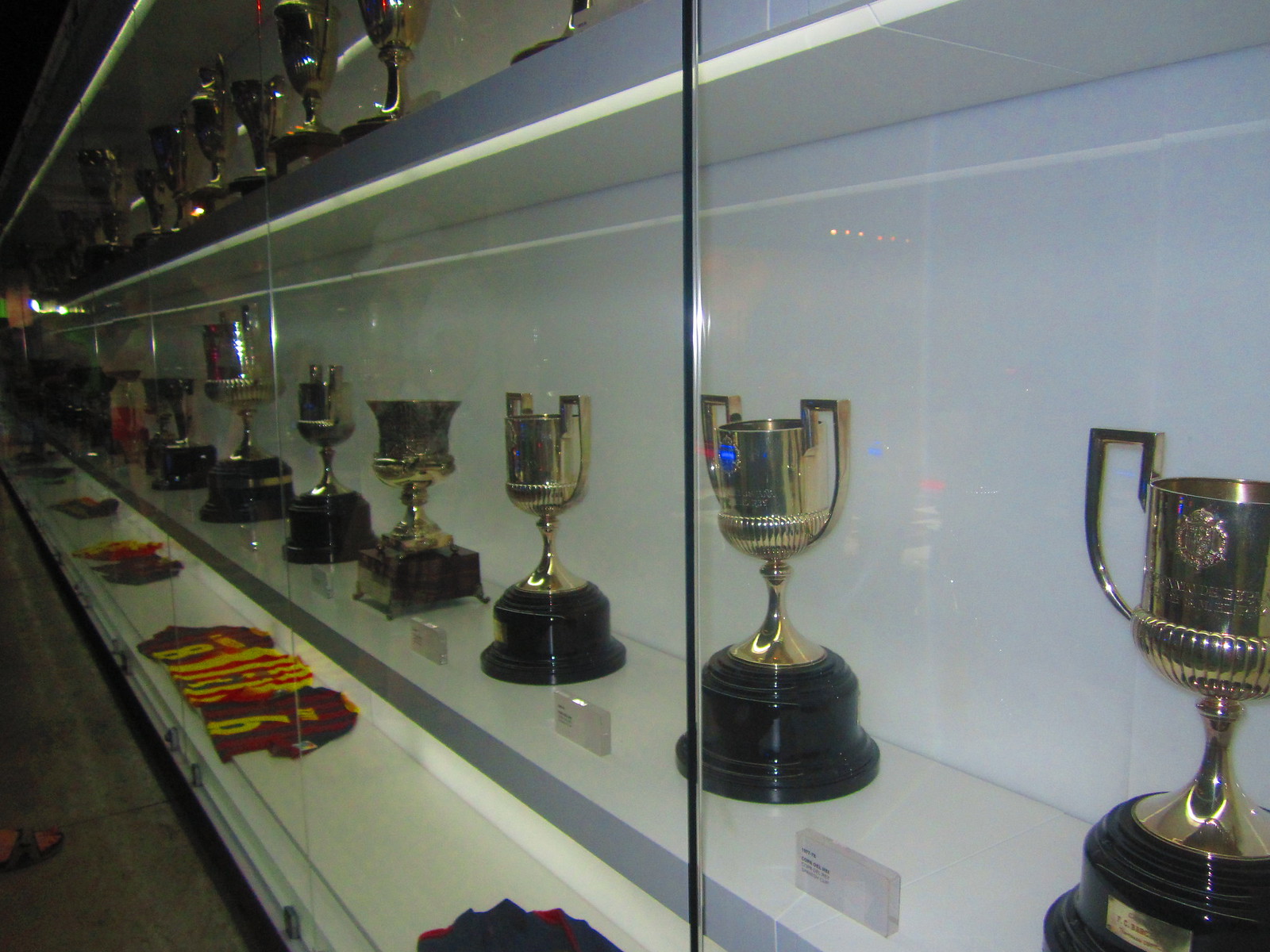The image depicts a large, glass-enclosed display case filled with numerous gold trophies arranged meticulously across multiple shelves. The angle of the photograph provides an expansive view, showing at least nine trophies on the middle shelf and several more on the top shelf. Each trophy sits on a black pedestal and features small acrylic plaques, presumably detailing the award's specifics, though the engravings are not legible from this angle. The bottom shelf contrasts with the middle and top shelves as it displays a collection of colorful soccer jerseys, neatly folded. Additionally, the photo captures a foot in a sandal, indicating that someone is observing the display, further suggesting the case is in a public setting, likely a school or a museum. Overall, the image conveys a clean and organized presentation of the trophies and jerseys.